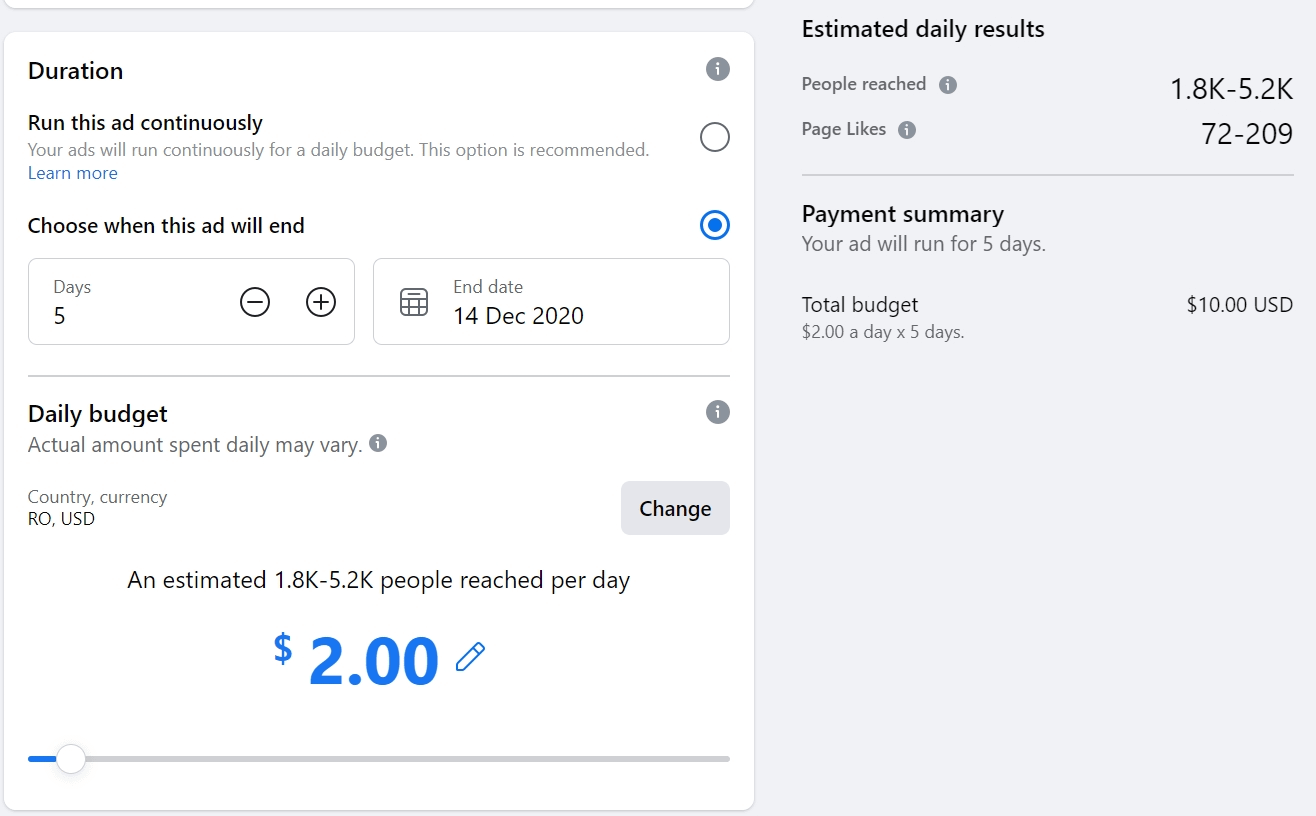**Caption:**

This image is a detailed screenshot of an ad purchasing page on a website, focusing on the duration and estimated daily totals sections.

In the upper left corner, the image is partially cropped, showing the bottom of a white box. Below this, there's another white box labeled "Duration" in bold black letters, accompanied by a grey eye icon to the right. Directly below, it displays the option to "Run this ad continuously" in small black letters, with an explanation that the ads will run continuously based on a daily budget—this is marked as the recommended option. Following this, there is a "Learn more" link in small blue letters, and a blank bubble to select this choice.

An alternative option, "Choose when this ad will end," is selected below. Here, a box labeled "Days" displays the number 5, with plus and minus signs available for adjusting the days. To the right, a date box marked "End Date" in grey shows "14th December 2020."

Towards the bottom left, it starts with "Daily Budget," under which it notes that the actual amount spent daily may vary, indicated by another grey eye icon. Below this is the "Country Currency," showing "ROUSD." Adjacent to this is a box labeled "Change." Below this, it states that an estimated 1.8 thousand to 5.2 thousand people will be reached per day with a $2 budget, visibly set by the large "$2" at the bottom. There is also a pencil icon to the right for adjustments, and a bar to modify the daily budget.

On the right side, it presents the "Estimated Daily Results" at the top in small black letters, followed by the metrics for "People Reached" and "Page Likes," displaying the respective amounts. Below these metrics, a "Payment Summary" section indicates that the ad will run for 5 days with a total budget of $2 per day, amounting to $10 USD in total.